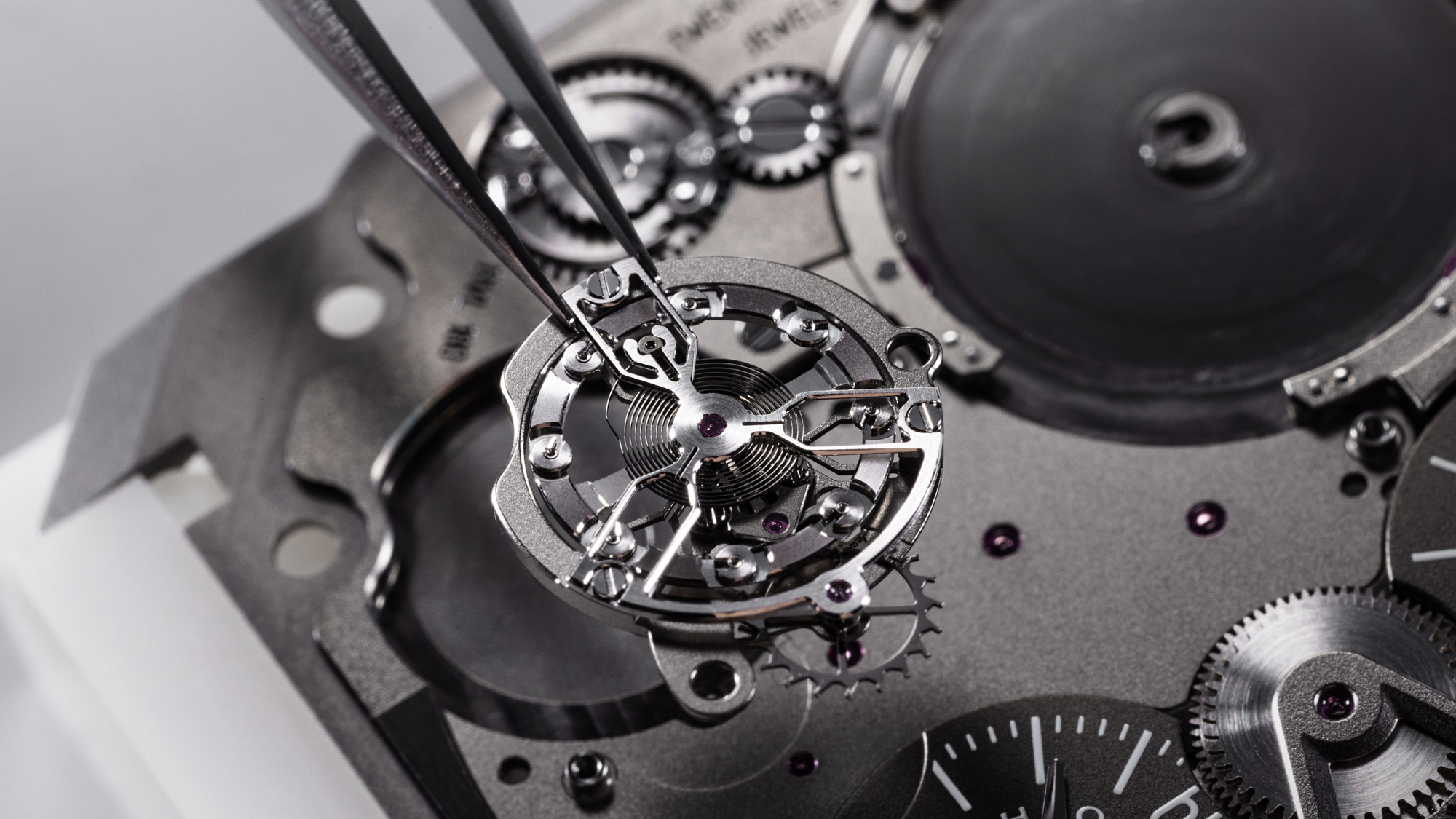The black and white photograph captures a high-resolution, crystal-clear image of a jeweler or clockmaker meticulously working on the interior of a watch. Dominating the foreground, a pair of professional-grade tweezers grips a delicate gear piece, which is part of the intricate clockwork. The scene is illuminated with such clarity that every individual component—gears, springs, screws, and frame—of the mechanical device is visible. The interior reveals a complex network of interconnected steel gears and springs, each playing a vital role in the function of the watch. Some writing, including the word "jewels", can be faintly discerned on the watch face, adding an element of authenticity and detail to the craftsmanship. The background remains slightly blurred, enhancing the focus on the tweezers and the gear they hold, further emphasizing the precision and meticulous nature of the clockmaker's work. The metal components, primarily made of aluminum and steel, contrast sharply against the light gray background, making the intricate details of the watch's inner workings stand out remarkably.